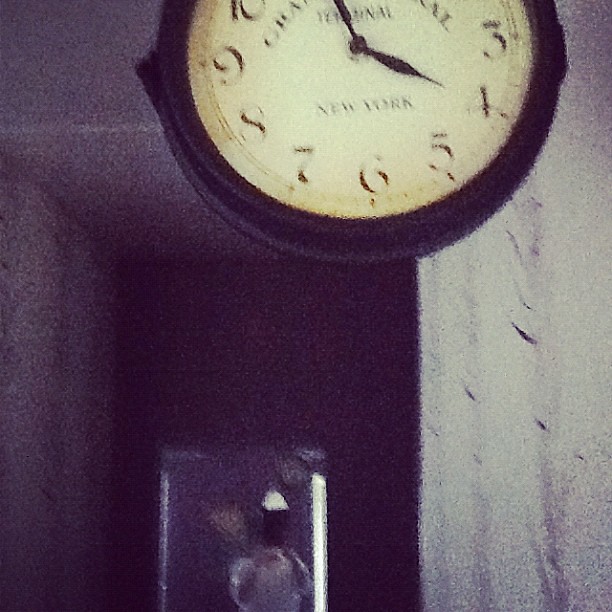In this blurry and grainy photograph, we see a clock prominently positioned at the top of the image, though its upper part is cut off. The clock displays the numbers 3 through 9, along with part of the number 10, all in Arabic numerals on a light face with a dark rim. The black hour hand points at 4, and the minute hand points between 11 and 12. Below the clock hands, the word "New York" is visible and the clock appears to tilt slightly to the left by about 5 to 10 degrees. Although difficult to discern due to the image's low quality, there is an indistinct curved text above the center, possibly saying "terminal," but it is mostly unreadable. The background features a dark area on the left and a white or light gray area on the right, which might suggest a hallway or room. Additionally, a small blurry black square is noticeable at the bottom edge of the photo, adding to the overall indistinct and enigmatic quality of the scene.